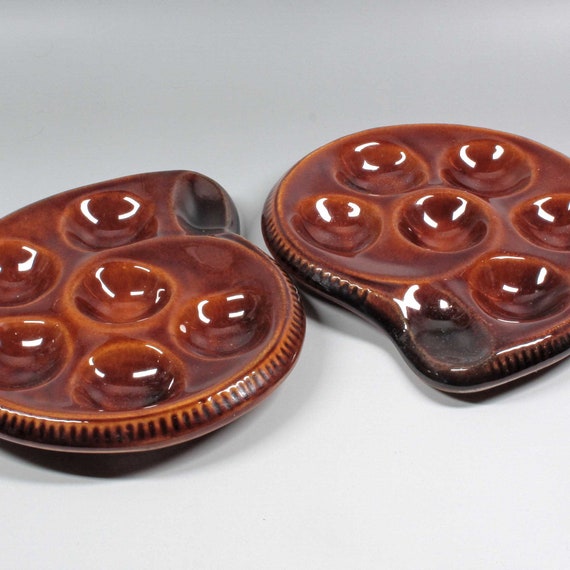This photograph showcases two identical ceramic trays, each with a glossy, glazed finish and an overall light brown to burnt orange-red hue, with darker brown or purplish edges. The trays have a unique spiral shell shape, bearing six circular indentations—resembling dimples—arranged in a snail-like pattern that could be used for holding small items, possibly for paints or deviled eggs. The ridged edges feature intricate lines, adding to their detailed craftsmanship. Each tray includes a small handling spot, enhancing their functionality. Set against a plain white background, sharp shadows cast by studio lighting highlight their polished, vintage appearance.